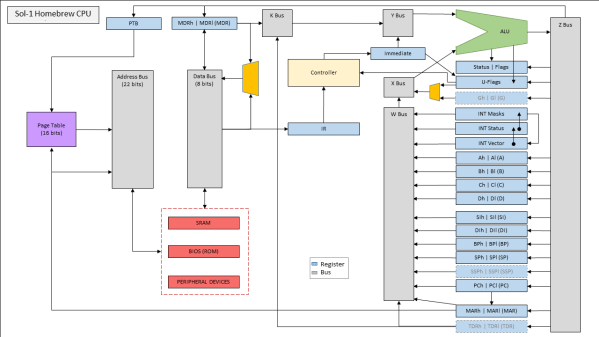This image is a detailed schematic of the Sol1 Homebrew CPU, illustrating the flow of data and the various components involved. At the top left, it’s labeled "SLL-1 Homebrew CPU." The diagram features a variety of colored shapes representing different elements: blue squares as registers, gray rectangles as buses, green shapes, and yellow shapes indicating various components and pathways.

Starting from the top, there’s a blue square labeled "ATB." It connects downward to a purple square on the left labeled "Page Table (16 bits)" and an address bus on the right labeled "Address Bus (22 bits)." Below these, an arrow points into a dotted square enclosing three rectangles labeled "SRAM," "BIOS (ROM)," and "Peripheral Devices." This dotted square shows communication through an 8-bit data bus connecting upwards to a gray square labeled "K Bus," which further connects right to the "Y Bus."

A black arrow indicates movement from a blue rectangle labeled "IR" towards the "Controller" inside a yellow square. From this point, instructions flow through an interconnected network of buses and registers. Notably, there’s a long gray rectangle labeled "W Bus" interfacing with smaller blue rectangles that detail various registers, including "Status," "U Flags," "INT Mass," "INT Status," "INT Vector," and "AH," "BH," "CH," "DH," with additional registers like "SH," "S," "PCI," "PC," and "MHMAR." The diagram ends at a tall gray rectangle labeled "Z Bus."

This comprehensive illustration represents the CPU’s architecture, detailing the pathways for data transfer and processing, highlighting the structure and interconnection of its components.